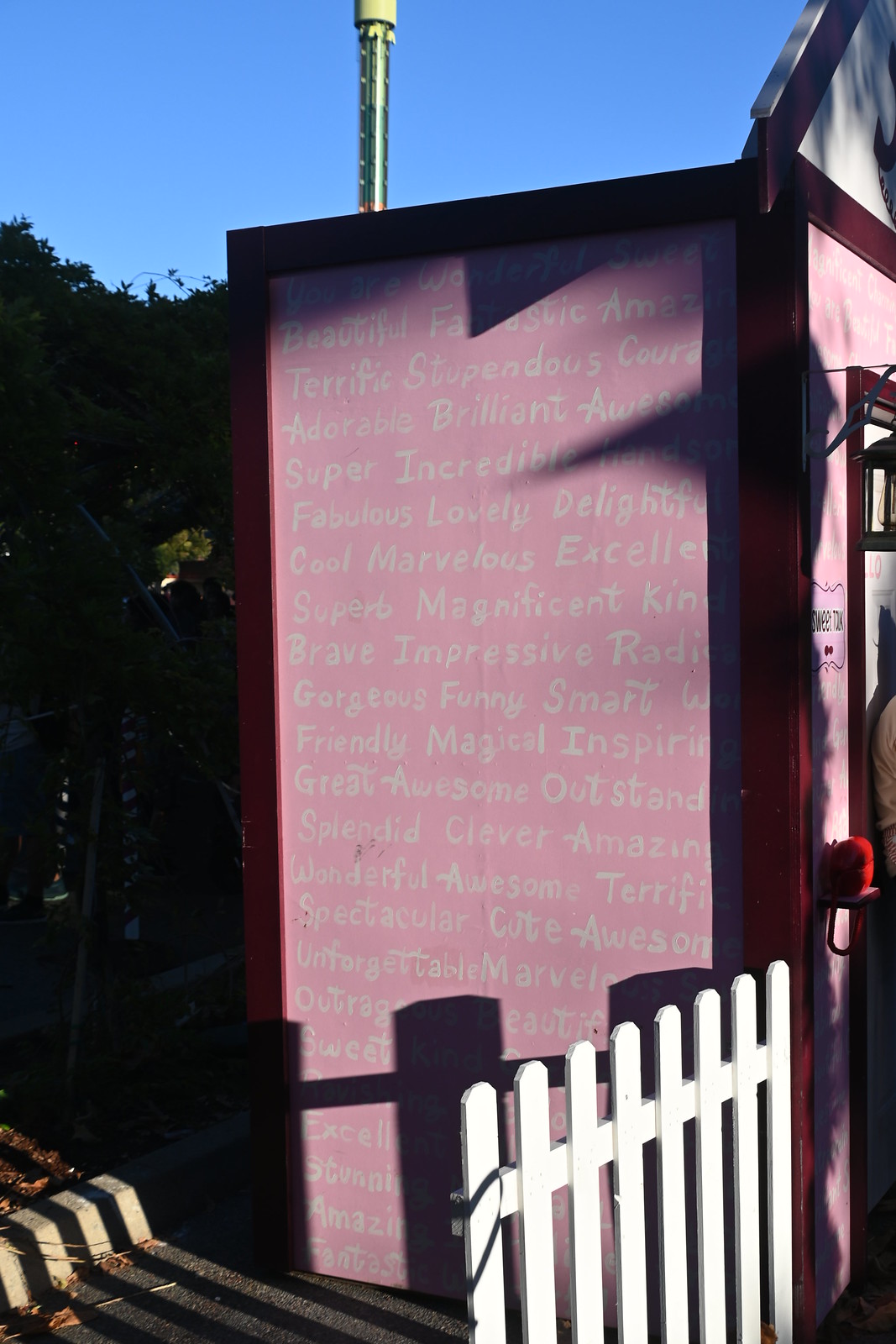This outdoor scene captures a large pink wall with a sturdy dark wooden border, standing next to a white picket fence. The sky is cloudy, adding a muted atmosphere to the vibrant structure, which could be an addendum to a building or a standalone shed. The pink wall is adorned with numerous positive reinforcement adjectives written in white letters. Among them are "Beautiful, Fantastic, Amazing, Terrific, Stupendous, Adorable, Brilliant, Super, Incredible, Fabulous, Lovely, Delightful, Cool, Marvelous, Excellent, Superb, Magnificent, Kind, Brave, Impressive, Gorgeous, Funny, Smart, Friendly, Magical, Inspirational, Great, Awesome, Outstanding, Splendid, Clever, Wonderful, Spectacular, Cute, and Unforgettable." The scene also features a wooded area in the background, hinting at a serene, somewhat residential setting. The pink wall stands on concrete, possibly near a street, with long shadows suggesting the photo was taken late in the evening or early morning.